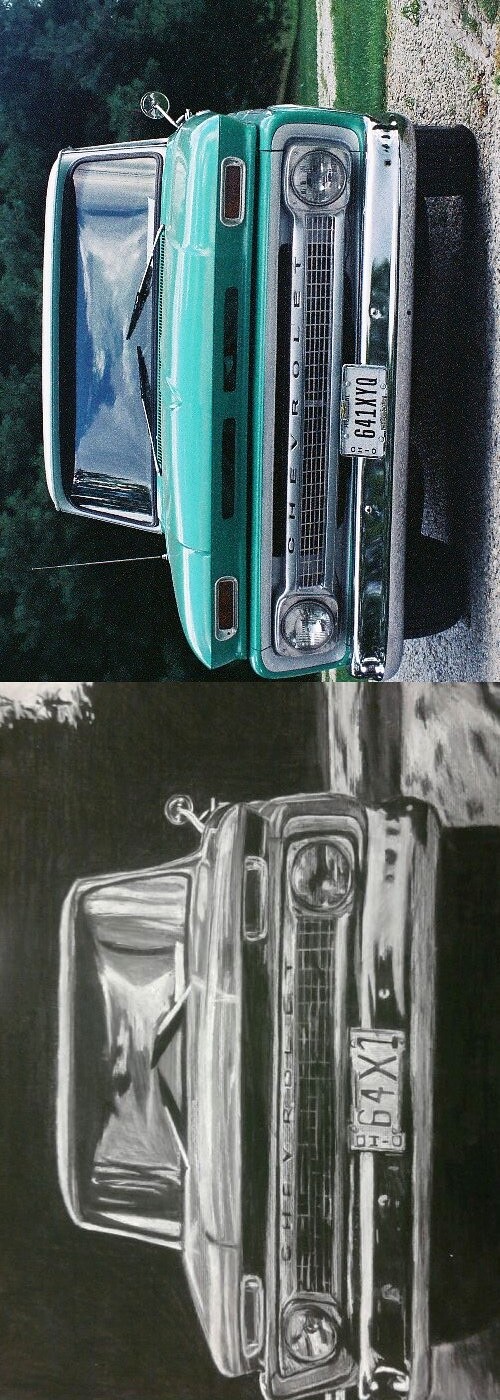The image is a vertically oriented, artistic depiction of a vintage truck, divided into two distinct sections. The top half showcases a digitally painted, color illustration of a classic seafoam green truck with a chrome bumper and a black and white license plate reading "64X1Y0." This section highlights detailed reflections on the chrome and glass, giving it a highly realistic appearance. The truck is seemingly parked on a gravel surface, with subtle hints of a natural background that includes trees. The bottom half of the image mirrors the top but in black and white, resembling a photorealistic digital drawing or filtered photograph. This monochromatic version retains the same details but emphasizes texture and contrast. Both sections are presented with a seamless transition, focusing primarily on the truck itself to create a cohesive and striking visual.